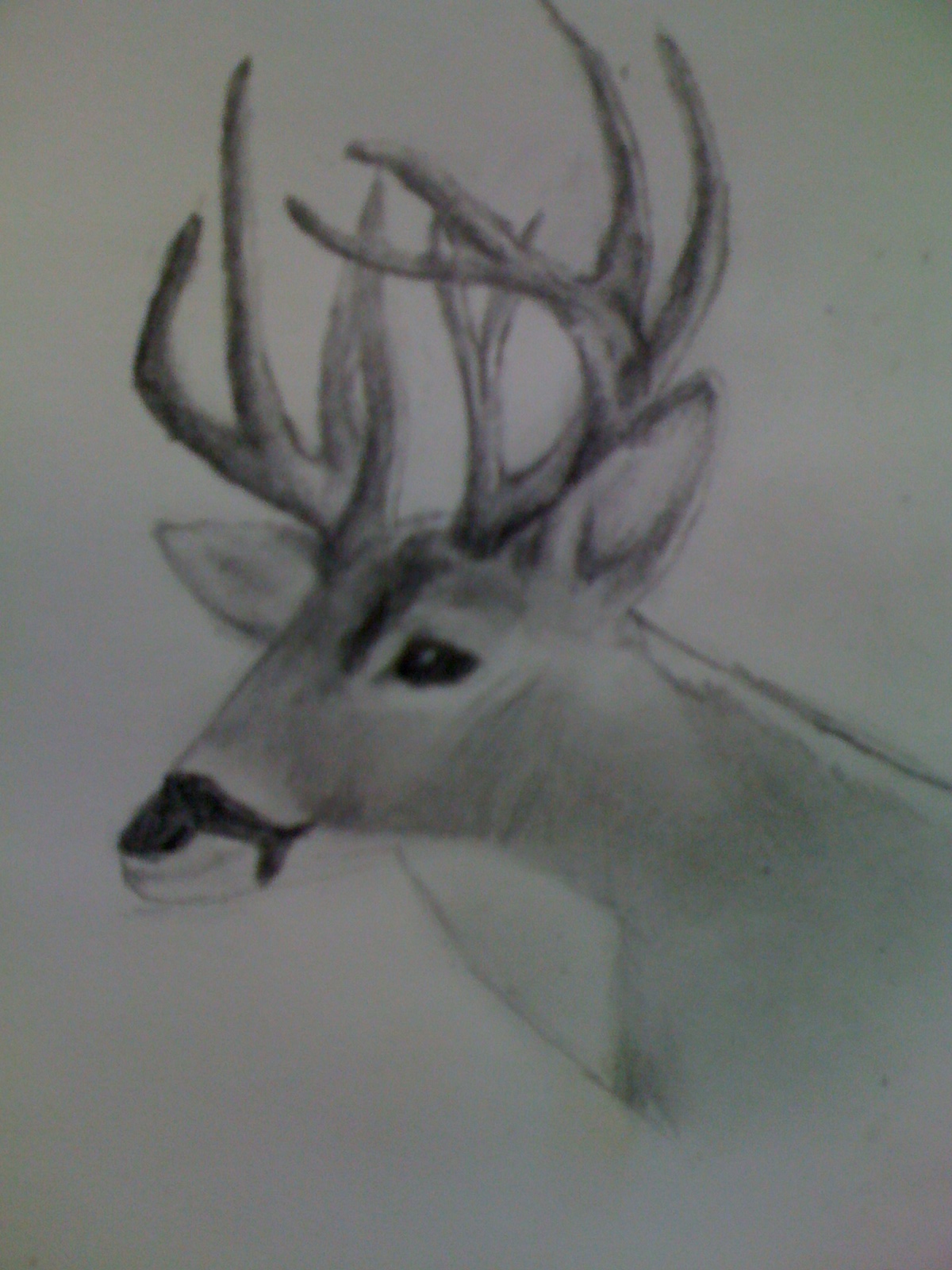This pencil sketch depicts the detailed portrait of a buck, a male deer, with a focus on distinct line work and shading. The drawing captures the texture of the deer's brown fur through meticulous shading, while the eyes and snout are artistically blackened out. Prominently, the buck displays an elaborate set of antlers, intricately drawn to exhibit their branching structure. The sketch includes the head and neck of the deer, emphasizing its natural grace and majesty. The artwork is rendered on a white background using dark grays and blacks, effectively highlighting the contours and definition in the deer's form. The level of detail in certain areas suggests a careful and deliberate approach, making this sketch a compelling study of a buck's features.